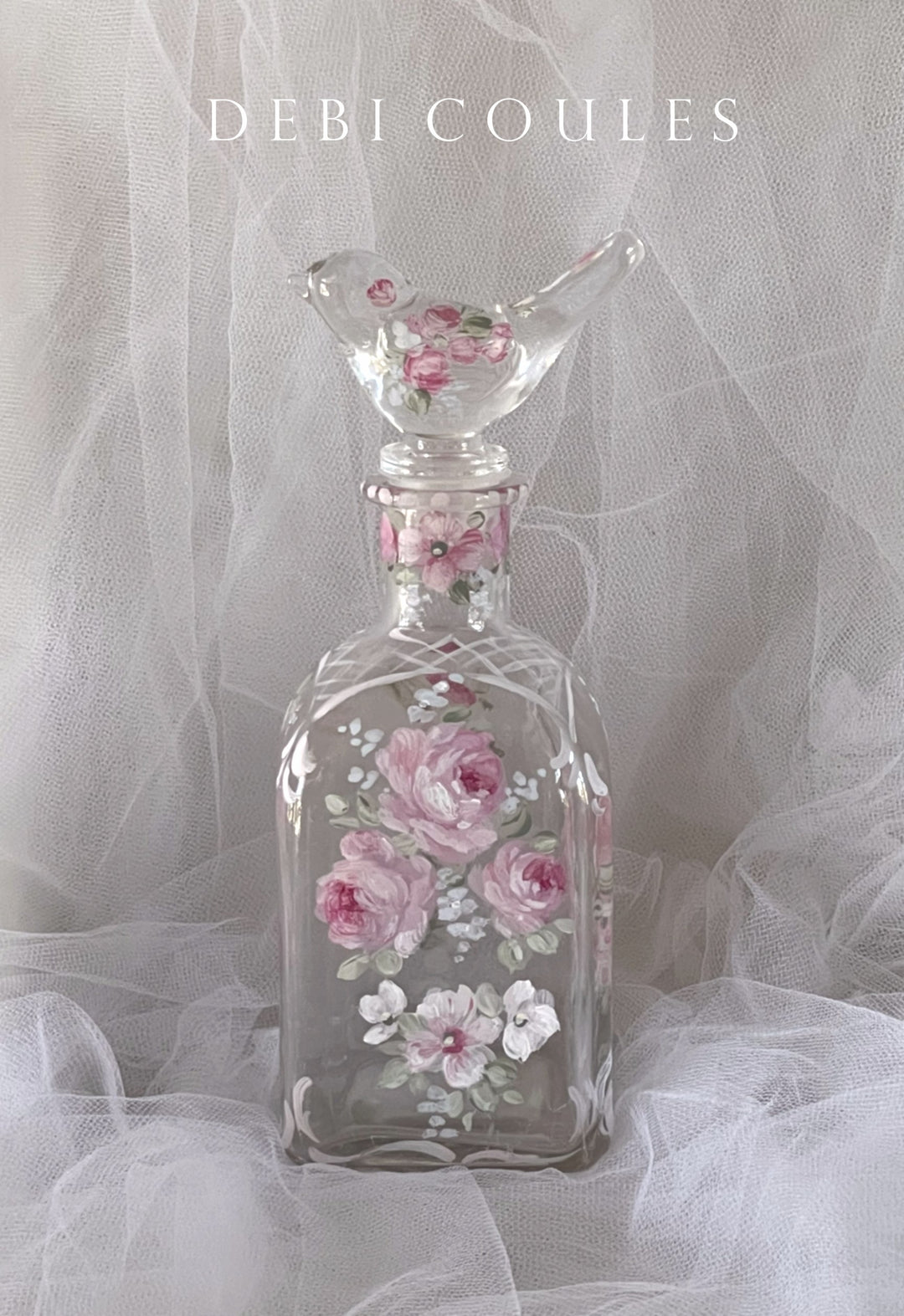This advertisement features a delicate and elegant glass bottle adorned with an intricate floral pattern. Set against a white background with draped, lacy netting, the scene exudes a sense of sophistication and charm. The bottle, branded with the name "Debi Coules" prominently displayed at the top in white text, showcases a design of pink and white flowers interspersed with touches of red roses. The glass stopper, sculpted into the shape of a small bird, mirrors the floral motif, adding a whimsical yet refined touch to the composition. The overall visual, with its harmonious blend of white lace and intricate swirls, creates a beautifully crafted and appealing advertisement.